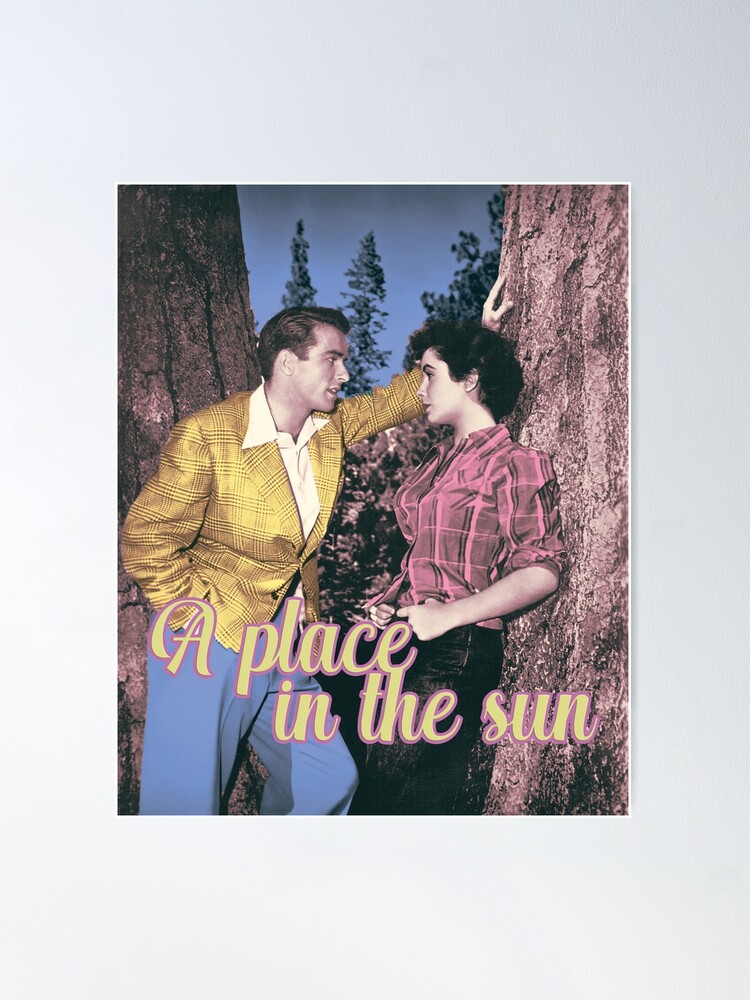This vintage photograph, possibly an advertisement for a book or play titled "A Place in the Sun," captures an intimate moment between a man and a woman in a forest. The woman, with short, curly dark hair and fair skin, leans against a tree. She is dressed in a pink plaid button-down shirt and black pants, with her hands resting at her waist as if hooked into her belt loops. The man, gazing intently into her eyes, has his right hand in his pocket and his left hand placed above her on the tree. He wears a white shirt, a gold plaid blazer, and light blue pants. The backdrop reveals a blue sky and several trees, adding to the nostalgic ambiance of the scene. The photograph, which appears to have been recoloured from an original black and white, features the title "A Place in the Sun" prominently in cursive lettering at the bottom, with yellow text outlined in red.